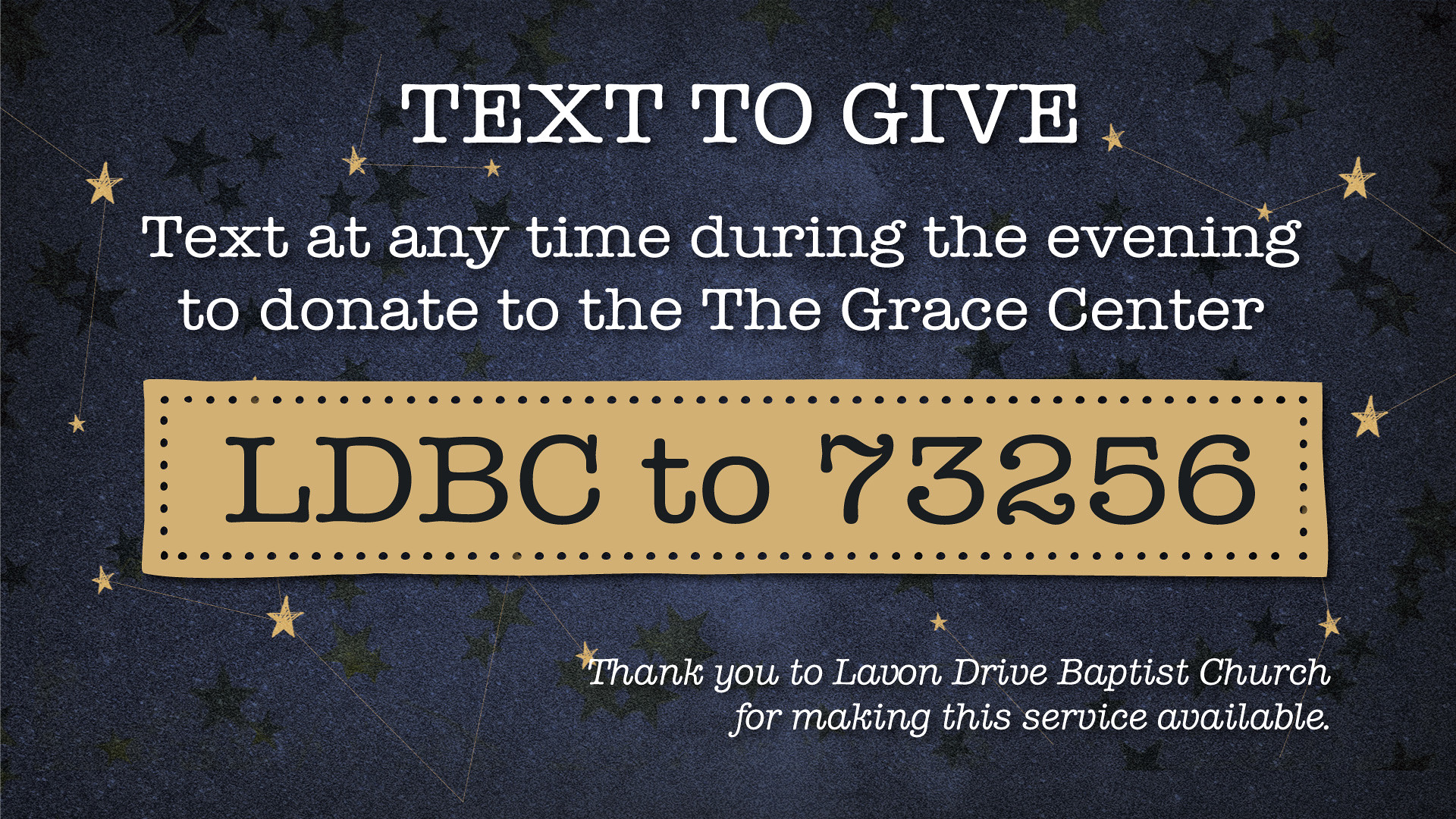The advertisement features a starry blue background adorned with beige and dark blue stars. Some stars are connected by delicate beige lines, resembling constellations. At the top, in bold white text, it reads "TEXT TO GIVE," followed by slightly smaller text that instructs, "Text at any time during the evening to donate to the Grace Center." Below this, there is a yellow text box with a black dotted border that contains the black text "LDBC273256." Beneath the yellow box, smaller white italicized letters express gratitude: "Thank you to Lavon Drive Baptist Church for making this service available." The blue background exhibits a granular texture in different shades, enhancing the celestial theme.